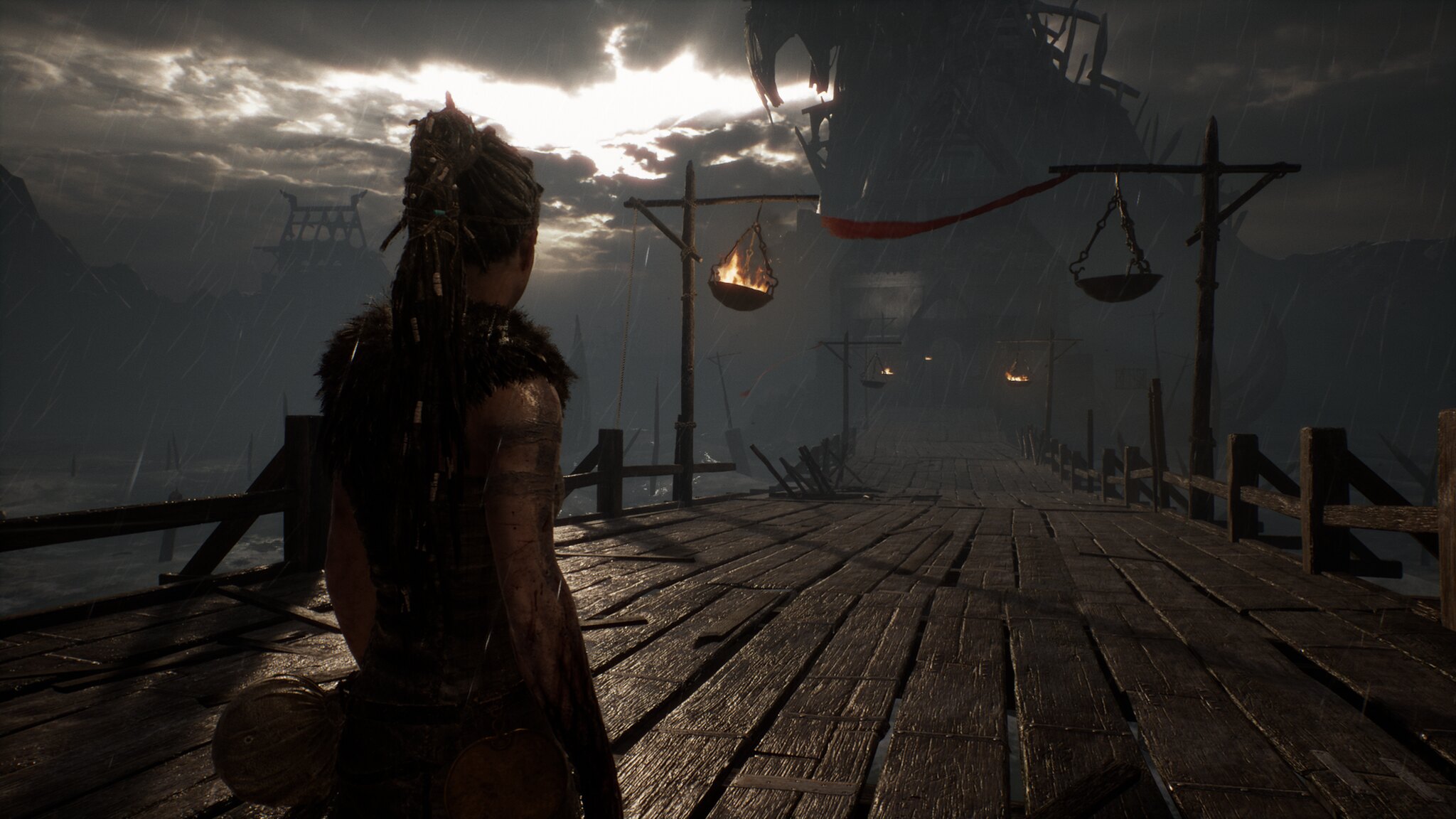A computer-generated image presents a mysterious and atmospheric scene. In the foreground, a man stands with his back to the viewer, shrouded mostly in shadow. His silhouette is outlined against a dimly lit backdrop, emphasizing his long hair, possibly styled in a top knot, and his shirt that leaves his arms bare. One of his arms is adorned with a leather strap, suggesting he may be carrying something that remains obscured by the darkness.

The setting is a lengthy wooden bridge that stretches into the distance, flanked by railings on either side. The bridge is enveloped in darkness, enhancing the enigmatic atmosphere. The sky above is overcast, with just a hint of sunlight struggling to penetrate the thick cloud cover, casting a muted light across the scene. 

Above the bridge, posts rise, supporting basins that serve as light sources. One of these basins contains a flickering fire, casting a warm, albeit faint, glow that becomes the primary source of illumination in this otherwise somber environment. The man gazes down the seemingly endless bridge, adding to the sense of mystery and intrigue that permeates the image.